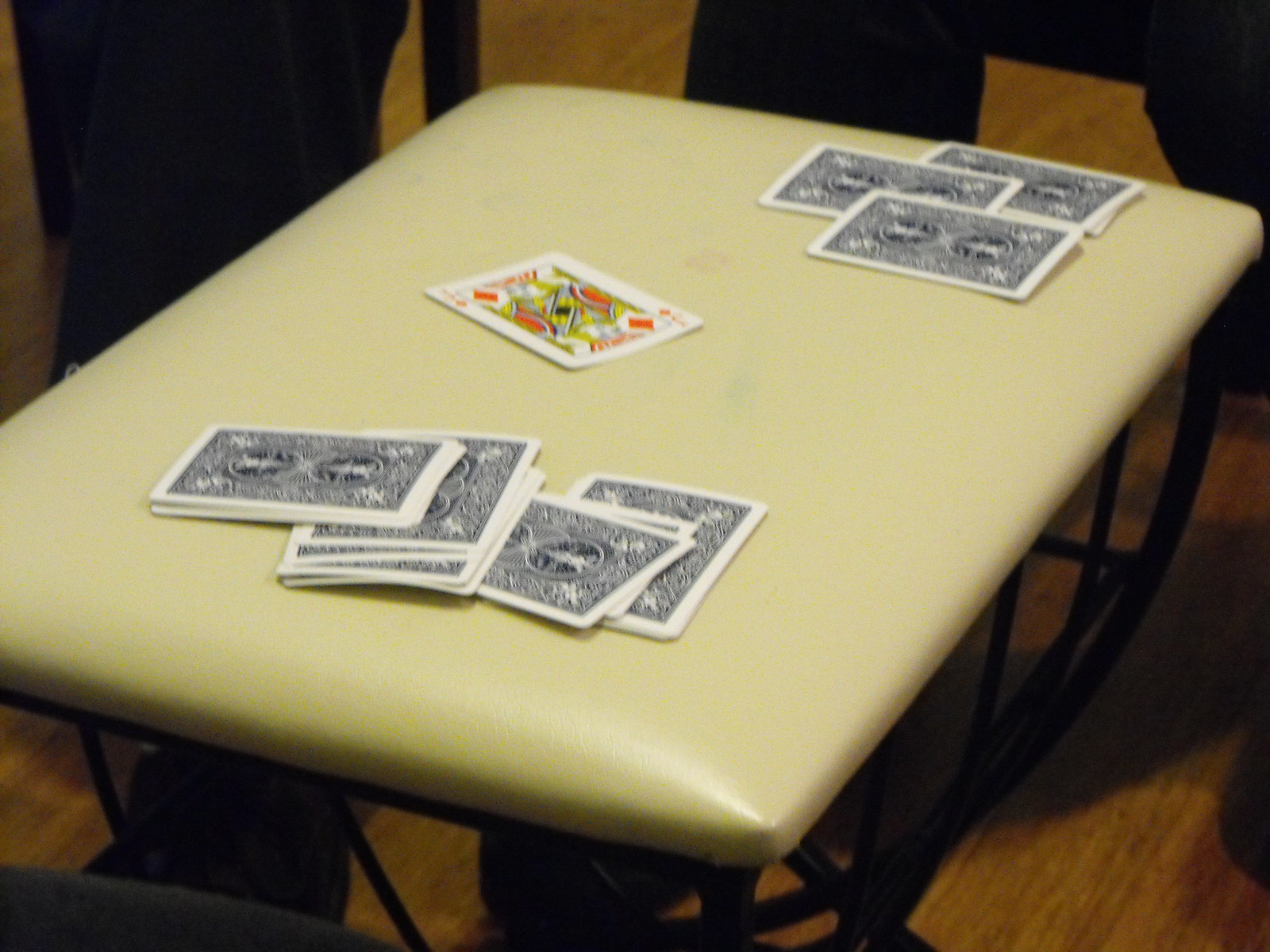The image showcases a white table set against a backdrop of a brown wooden floor. Visible around the table are black chairs and the black legs of the table itself. Scattered on the white surface are several playing cards. At the top of the table, three cards are flipped over, revealing their blue backs, while towards the front, a pile of additional cards also lies face down, concealing their identities. Dominating the center of the table is a single card, the Jack of Diamonds, prominently displaying its vibrant colors amid the other face-down cards. The composition draws attention to the game in progress, hinting at an engaging moment in gameplay.